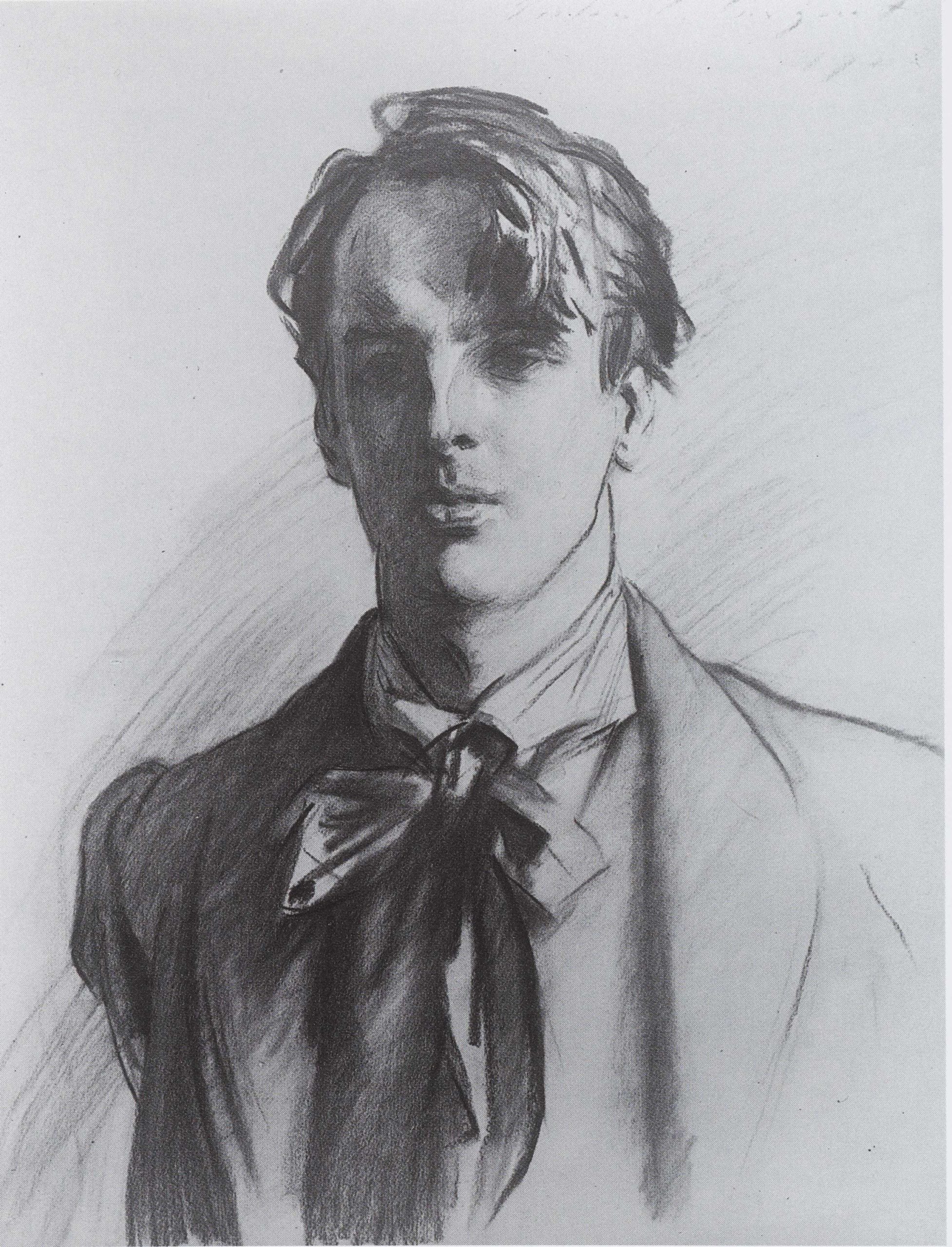A detailed black and white pencil sketch depicts a distinguished young man, exuding an air of high class and era-specific style. The man features a sharp jawline, full but defined lips, and bushy eyebrows. His short hair, slightly curled at the front, adds to his sophisticated appearance. He dons a fancy suit with a high-collared shirt and a broad, old-fashioned jacket that suggests late 18th to early 20th-century fashion. Completing his elegant attire is a loose and long bow tie. While only his upper body is visible, the precision in the sketch highlights his distinguished look, reminiscent of a figure one might find in historical art or literature.